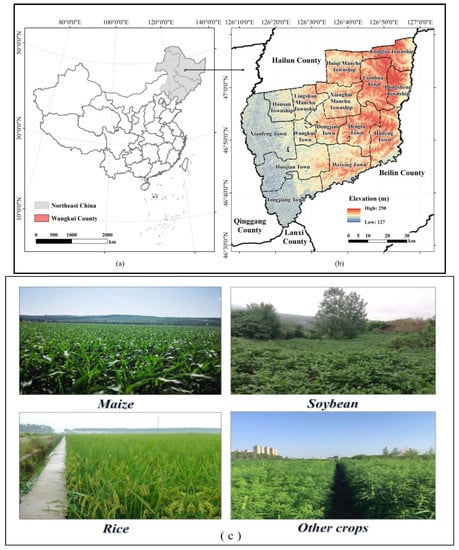The image showcases a detailed and informative layout focusing on agricultural and geographical features of Northeast China. The top section contains two adjacent maps: the left map is a sketched, black-and-white rendition labeled "Northeast China," specifically highlighting Wenquai County. It is a minimalist map featuring county outlines with basic grayscale shading at the top right corner. The right map, labeled "Northeast China," is a colorized elevation map detailing various counties and towns, including Kuning County, Beilin County, and Hailun County. This map shows elevation ranging from 127 to 290 meters and is marked with coordinates on the top and sides, labeled A on the left and B on the right.

The bottom section of the image features four photographs of different crops commonly grown in the region. The top left photograph is labeled "maize," depicting lush green fields of maize with a faint bluish mountain in the distance. To its right is a photograph labeled "soybean," showing a field of soybeans with some trees interspersed. The bottom left image, labeled "rice," shows a vast, flat area of rice fields with a large stream running through it. The bottom right photograph, labeled "other crops," presents a diverse green landscape with tall buildings visible in the far distance on both the left and right sides. This photograph is further labeled as C.

Together, these maps and photographs provide a comprehensive view of the agricultural landscape and geographical context of Northeast China.